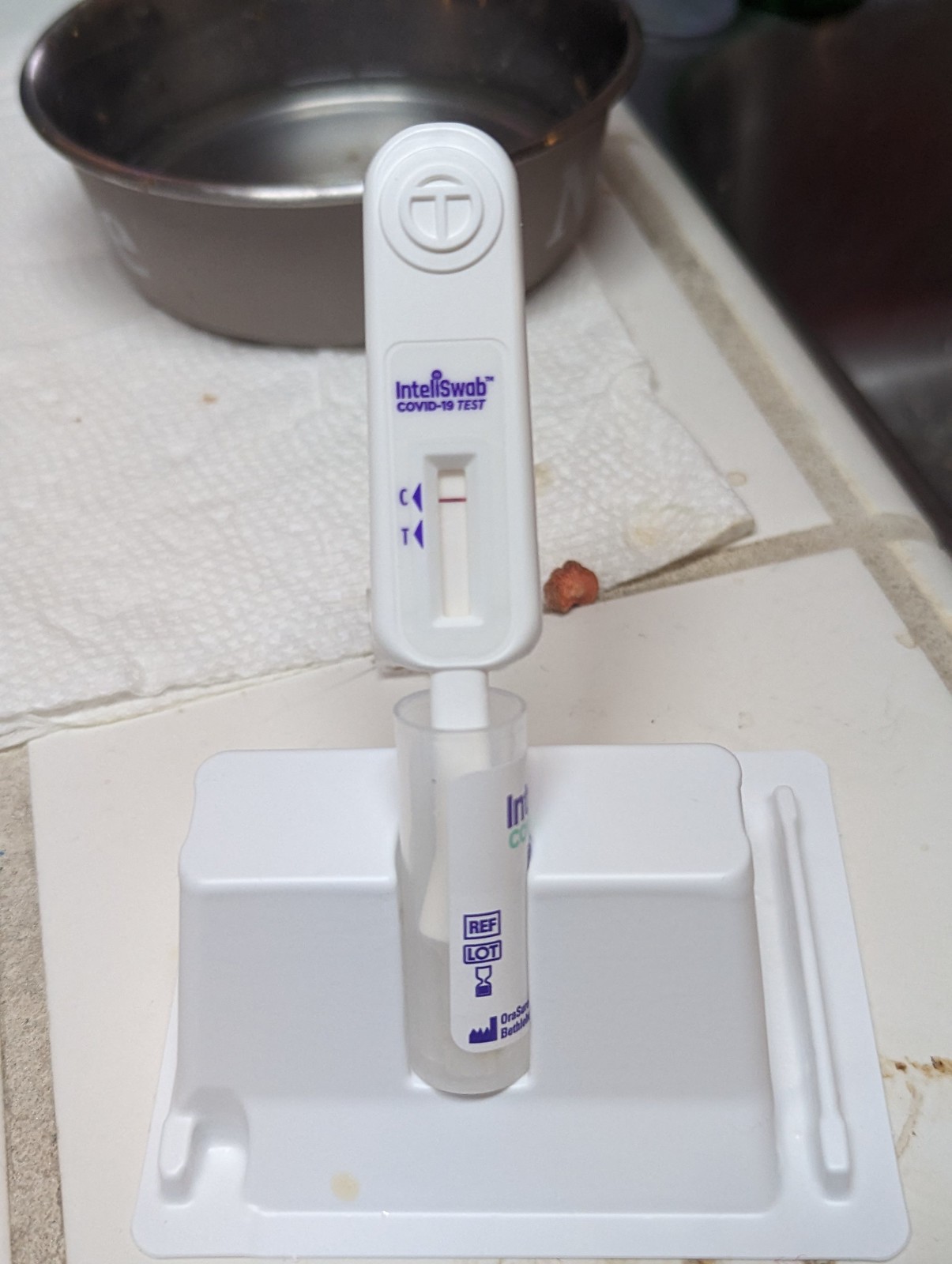A detailed photograph showcases a COVID-19 test setup, arranged on a white tile surface with grout that appears grayish and slightly dirty. The test itself is slightly tilted to the left. Behind the test, placed on the tile counter, is a round silver bowl resting on a folded white paper towel. A round red object is visible on the left side of the paper towel, centered in the image.

In the foreground, the COVID-19 test is presented in a unique cube-like, though more rectangular, base. The base flares out into a square shape and supports a clear cylindrical test tube. From the top of the test tube protrudes a long, oval-shaped white plastic device. The device bears the inscription "Inteliswab COVID-19 Test" prominently in the center. It features a vertically oriented rectangular indented opening with a red line crossing the top. To the side of this opening are the letters "C" and "T," denoting the control and test lines respectively.